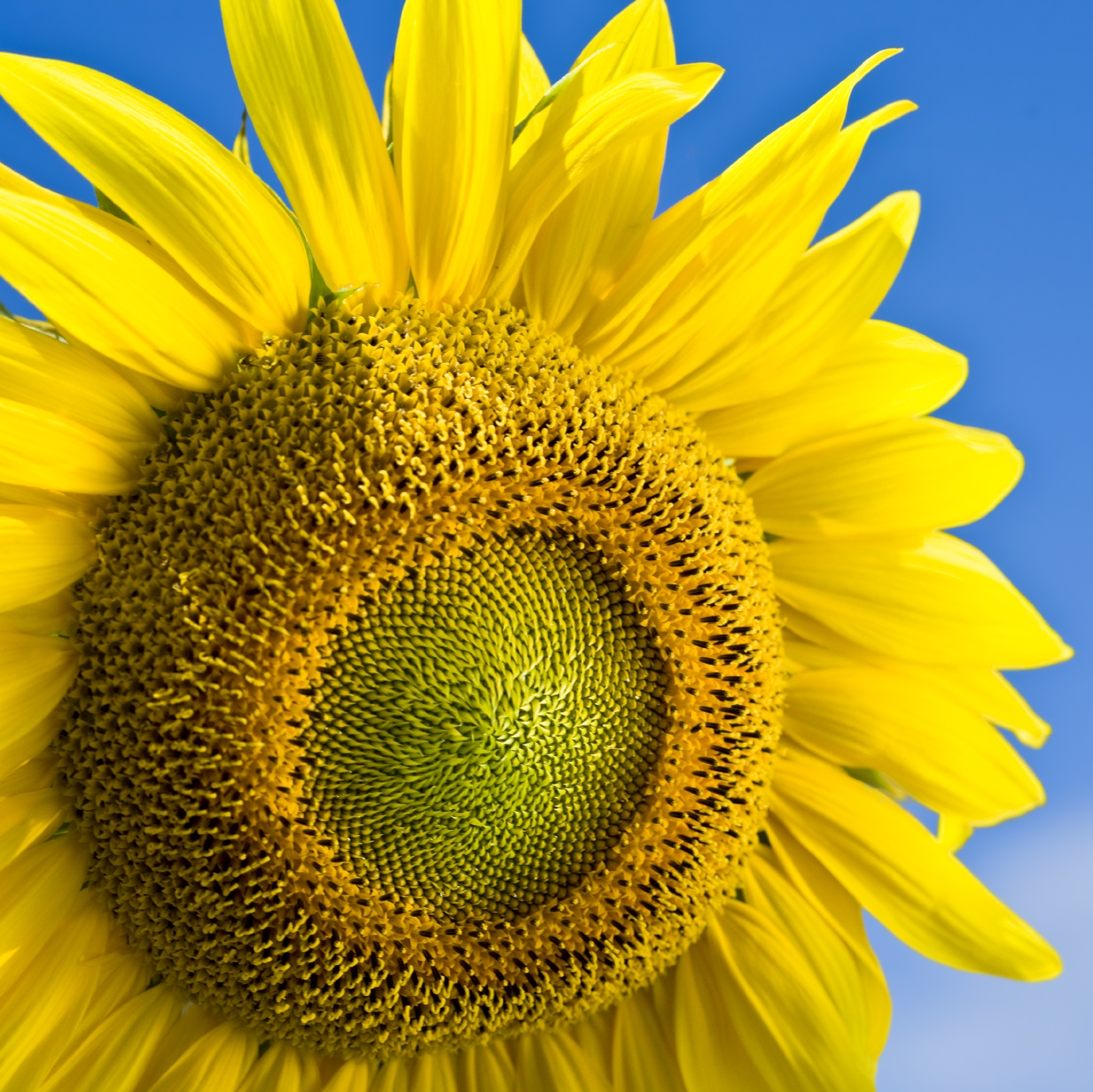This close-up photograph captures the vibrant beauty of a sunflower in exquisite detail. The flower, with its bright yellow petals, takes up nearly the entire frame, extending beyond the left and bottom edges. Set against a bright cerulean blue sky with wispy clouds visible towards the bottom right, the photograph emphasizes the stunning contrast between the sunflower and its vivid background. The sunflower's intricate center transitions from a yellow edge into a green-yellow inner ring. The outermost part of the center features a detailed honeycomb-like pattern, gradually darkening into bright orange before shifting to a longer, thistle-like green at the core. The outdoor setting and high-definition quality of the image highlight the photorealistic textures and shades, with sunlight illuminating the right side and casting shadows on the left. No text is present, allowing the natural elements and colors to take precedence.